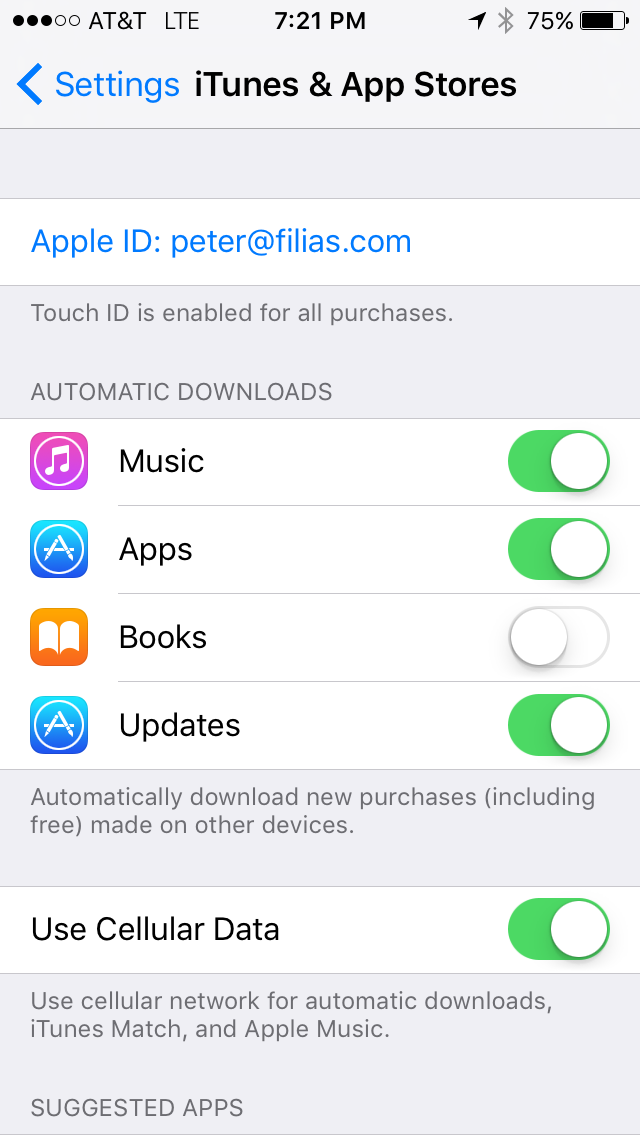This is a screenshot of an iPhone's iTunes and App Store settings, captured at 7:21 PM with AT&T as the carrier. The phone battery is at 75%. The background of the settings screen is primarily gray with blue and black text. At the top, it shows the Settings and iTunes & App Stores options. The Apple ID displayed is peter@filias.com. Touch ID is enabled for all purchases. Under Automatic Downloads, the settings for Music, Apps, and Updates are activated (with green toggles), while Books is deactivated (grayed out). A note indicates that new purchases, including free ones from other devices, are set to download automatically. The Use Cellular Data option is turned on, allowing automatic downloads, iTunes Match, and Apple Music to use the cellular network. The section for Suggested Apps appears at the bottom, trailing off the screen.